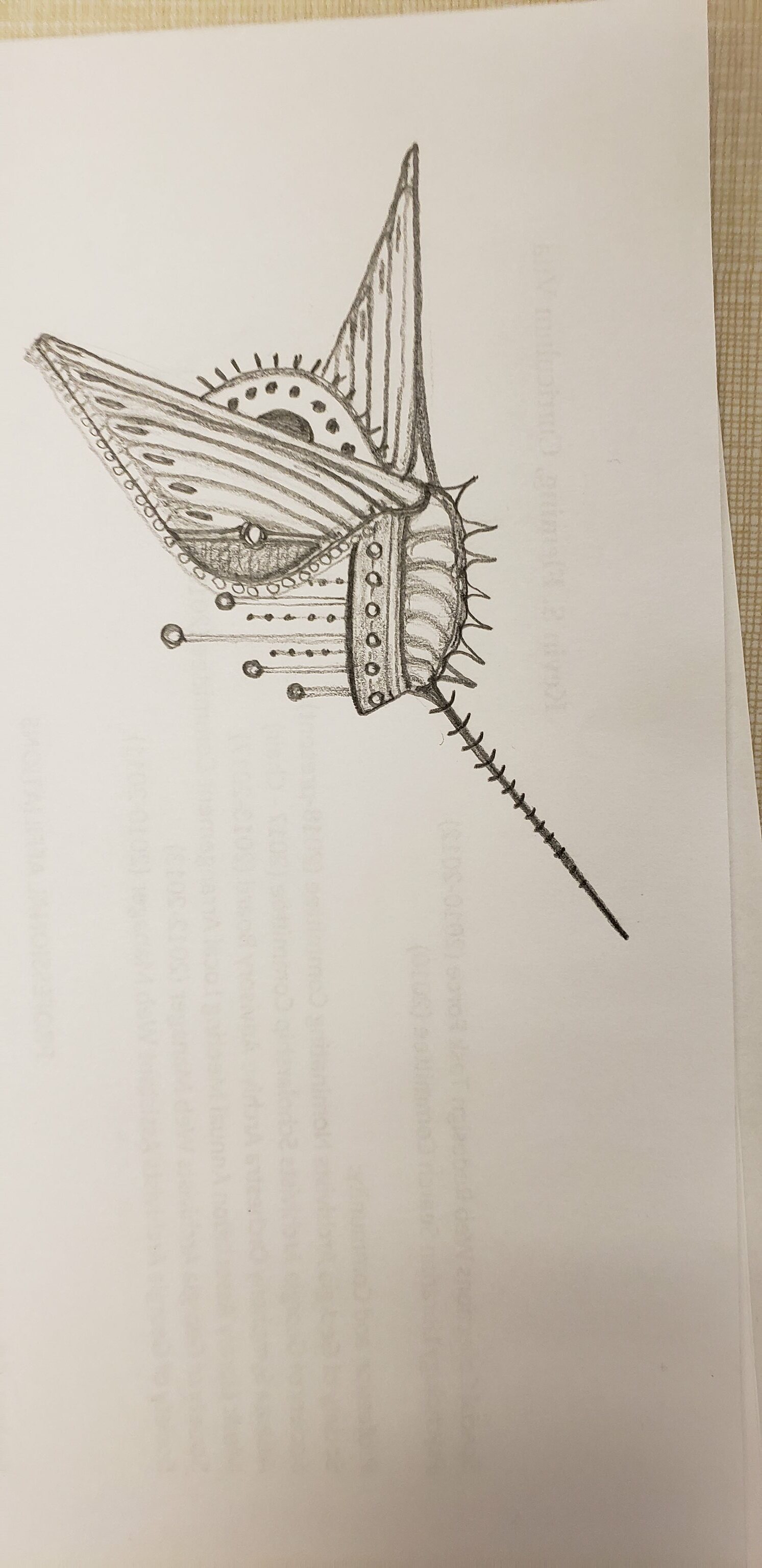This image showcases an intricate pen and ink or charcoal rendering of an enigmatic object, meticulously drawn on a piece of pristine white paper. The object itself, assembled from multiple components, features an elongated proglossus at its front, adorned with bands that gracefully curve from a wider base to a narrower top. The level of detail in the drawing is remarkable, with ornate techniques such as hatching, cross-hatching, and shading creating textures and patterns throughout the object. Additional decorative elements include small open circles, jagged edges, vertical and horizontal lines, and various other intricate details. Faint shadows at the bottom of the paper hint at underlying text, though it remains indiscernible and subtly shines through the surface. The paper rests on a brown, grass-cloth type surface, adding to the drawing's organic and tactile presentation. Despite its elaborate detail, the object remains unidentifiable, existing purely as a creation of artistic imagination.